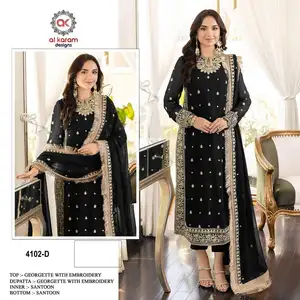The image features a model, likely an Indian woman, presented in two adjacent photographs as if from a magazine spread. She is elegantly dressed in a black and gold outfit that resembles either Indian or Arabic royal attire. The ensemble includes long, dangly earrings, and she has dark hair. There is detailed embroidery and beadwork around the neck, wrists, and the central part of the dress, and it is complemented by a luxurious cape lined with soft fur on one side, which can be draped over her arms. 

In the left photograph, she is shown draping the cape. The image is labeled with "4102-D" in the bottom left corner, and text at the top mentions "Al-Karam Designs" and "top, Georgette with embroidery, inner santun, bottom santun," although some of this text is blurry. The right photograph presents the model from a different angle, emphasizing the intricate details of the outfit.